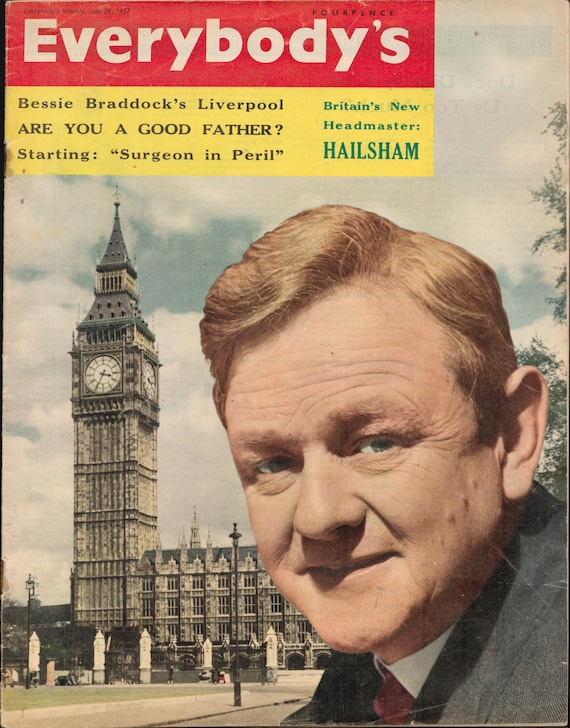The cover of a vintage magazine titled "Everybody's" prominently features an older gentleman with reddish-blond hair, blue-green eyes, and a distinctive series of three bumps on his left cheek. He is smartly dressed in a suit with a black collar, a barely visible white inner shirt, and a red tie, giving him a distinguished appearance. His expression is marked by a slightly raised eyebrow, a thin mouth forming a half-smile, and noticeably large ears. 

The background prominently showcases London's iconic Big Ben and the Houses of Parliament against a cloudy sky, hinting at the magazine's British origin. 

In the top left corner, the date reads "June 29th, 1957," and "Fourpence" is noted in small black text, indicating the magazine's price. The top of the magazine features a red banner with the title "Everybody's" in bold white letters. Below this, a yellow box contains headlines in black and green text: "Bessie Braddock's Liverpool," "Are You a Good Father?" "Starting: Surgeon in Peril," and "Britain's New Headmaster, Hailsham." This old, well-preserved magazine cover combines the elegance of its era with a snapshot of contemporary societal concerns.